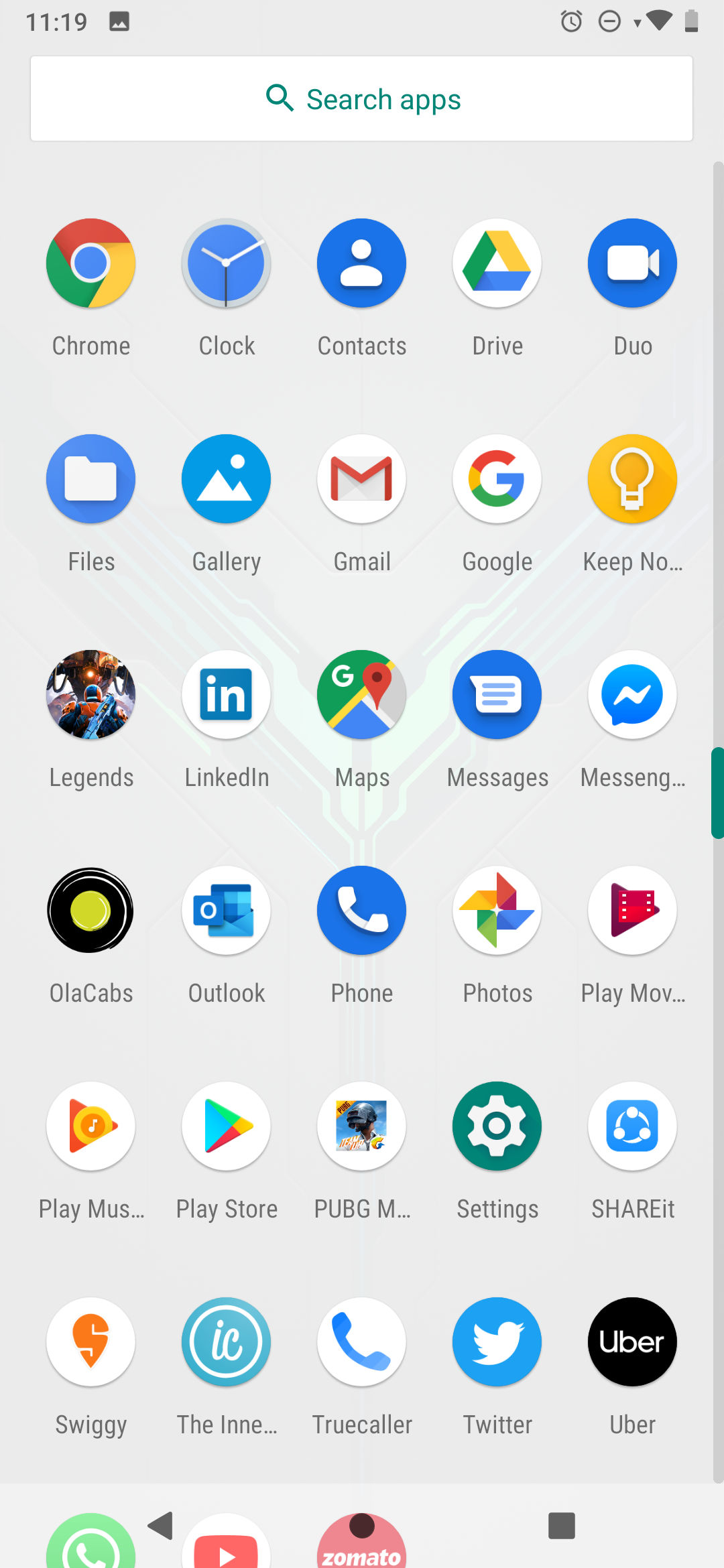This image depicts a smartphone home screen with a variety of application icons arranged in multiple rows. The time displayed in the upper left corner is 11:19, accompanied by a small square icon. To the right, there is a battery indicator showing very low charge, represented by a thin black line near the bottom. At the top of the screen, there is a white search bar with a green magnifying glass icon, labeled "Search apps."

The app icons are organized into several rows. The first row features icons for Chrome, Clock, Contacts, Drive, and Duo. The second row includes Files, Gallery, Gmail, Google, Keep, and Note. The third row contains Legends, LinkedIn, Maps, Messages, and Messenger. The fourth row starts with an app represented by a black circle with a neon green circle inside, followed by Ola Cabs, Outlook, Phone (depicted by a blue circle with a white telephone inside), Photos, and Play Movies. 

In the next row, the icons are for Play Music, Play Store, PUBG, Settings (a green circle with a white gear), and an app represented by a white circle with a blue square inside, labeled Share It. The final row consists of Swiggy, INNE, Truecaller, Twitter (depicted by a blue circle with a small white bird inside), and Uber (inside a black circle with the word "Uber").